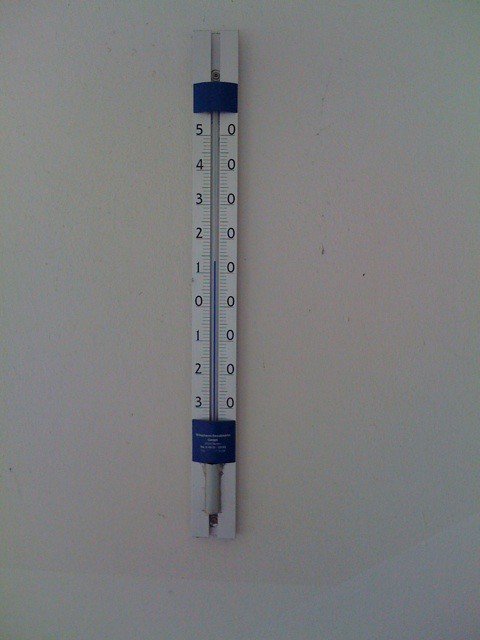The image features an old-fashioned thermometer, which appears to be either hanging on a wall or lying on a floor. The thermometer itself is mounted against a white background, which transitions into a peachy, shaded area at the bottom. This transition is marked by horizontal and diagonal lines that separate the white section from the shaded area.

The thermometer contains a blue liquid, which rises to just over the 1.5 mark. The temperature scale on the thermometer starts at 0 and ascends in increments, marked as 0, 1, 2, 3, 4, and 5, with all 0s listed along the right side.

The device features a blue label at its base, and a blue band at the top that appears to secure the glass part of the thermometer to its white housing. Despite some writing at the bottom of the thermometer, it is difficult to read. Moreover, the image obscures the exact end of the device, partly due to some paint covering the lower section, contributing to its rather generic appearance.